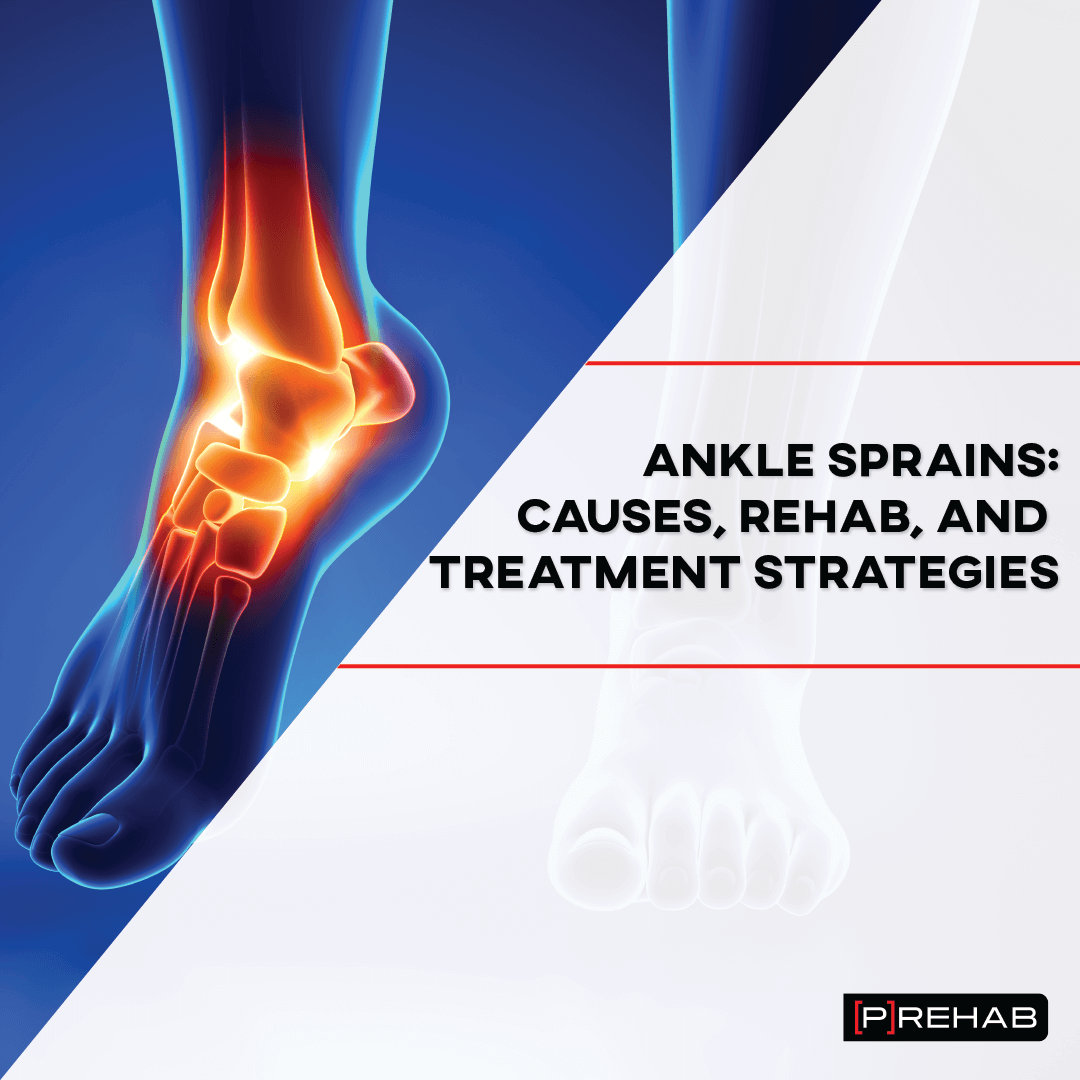The image is a detailed leaflet about ankle sprains, their causes, rehabilitation, and treatment strategies. The design features a blue-toned graphic of an ankle with an inflamed area highlighted in orange and red to signify injury. This graphic is positioned in the upper left corner, occupying about 20% of the space. The background transitions from blue in the top left to white in the remaining space, with a faint watermark of the same ankle graphic. On the right side, there are two vertical lines extending to the edge, with text in black reading "ankle sprains causes rehab and treatment strategies." In the bottom right corner, a black rectangle contains the word "P-R-E-H-A-B," with red brackets around the letter 'P'.